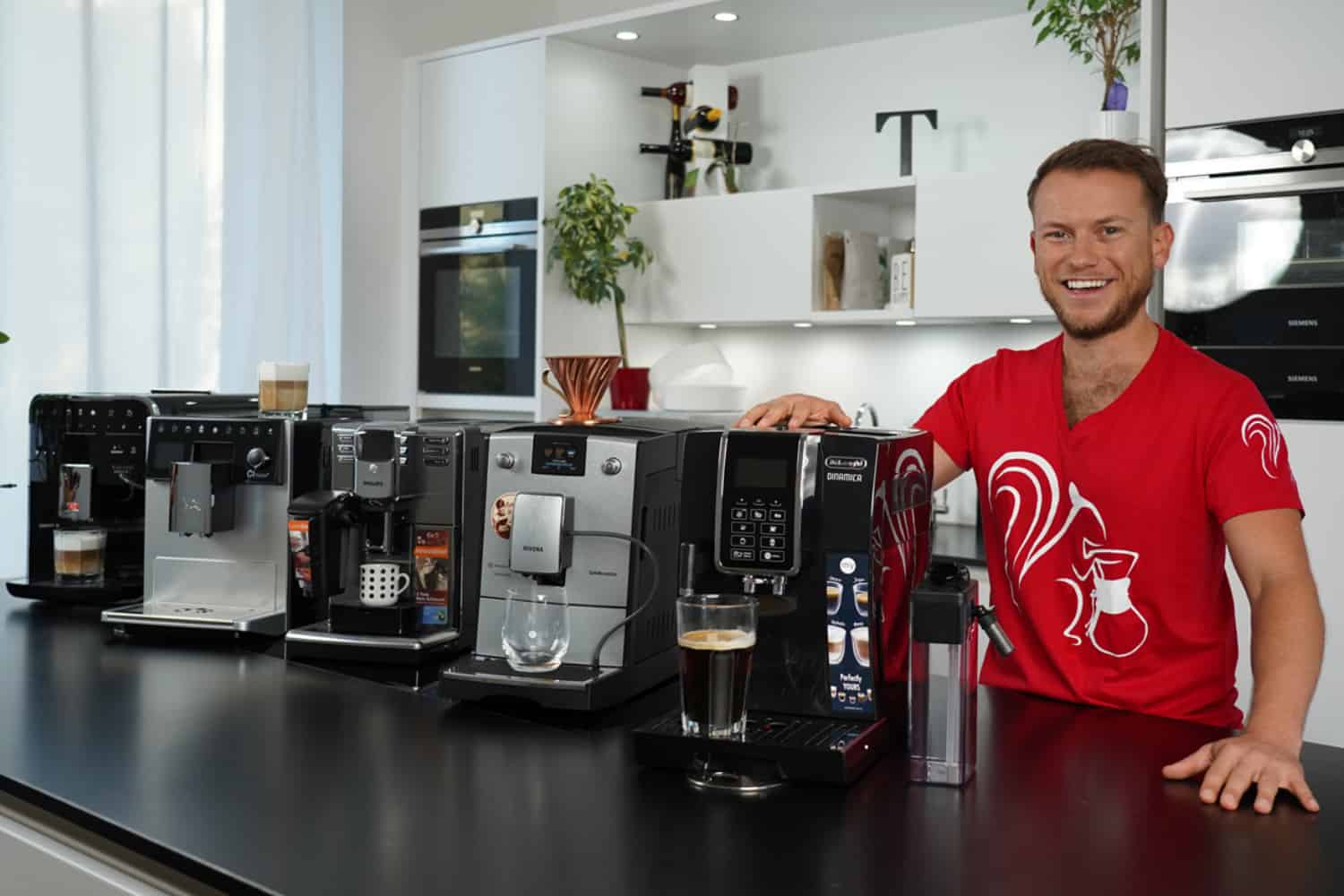This detailed photograph captures a sleek, modern kitchen where a smiling man in a bright red t-shirt adorned with a white squirrel logo proudly showcases an array of high-end coffee-making equipment. He stands behind a large, black-topped kitchen island, with various advanced coffee devices arrayed meticulously in front of him. From left to right, the lineup includes a modern square French press, a black espresso machine, a silver drip coffee maker, a gray-ish cappuccino machine, and another bulky coffee maker. The countertop features glasses and coffee mugs ready to catch freshly brewed coffee. The backdrop reveals a sophisticated kitchen setting with built-in appliances, a wall oven, an open shelf with a vase of greenery and a decorative letter T, a small freestanding wine rack holding three or four bottles, and another built-in appliance. The overall scene exudes a sense of pride and expertise in coffee brewing, reflecting the man's role as either a purveyor of coffee or an enthusiastic advocate of coffee-making equipment.